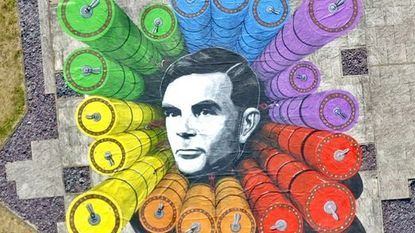The artwork is a horizontal rectangle, wider than it is tall, featuring a detailed and vibrant composition. At the center is a man's head rendered in black and white, with dark hair parted to his left and a pale complexion. He gazes slightly to the left rather than directly forward. Surrounding his monochromatic face is a striking arrangement of tubular, cylinder-type objects, segmented and stacked in groups of three. These colorful tubes form a circular pattern starting from the upper left corner and progressing clockwise. Beginning with three green tubes, followed by three blue, three purple, three red, three orange, and finally three yellow tubes, the colors are reminiscent of the rainbow spectrum. This colorful array contrasts vividly with the man’s black and white portrait. The background consists of various shades of gray tiles, with a patch of pea green to the left, adding an additional layer of visual interest to the compelling and eclectic image.